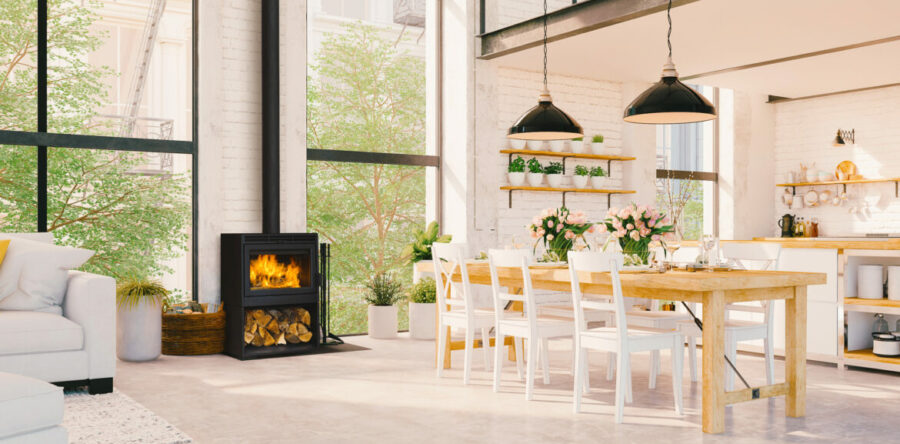The spacious, high-walled great room, painted predominantly white, exudes a modern, minimalistic vibe with its carefully curated furnishings. Dominating one wall is a black, traditional wood-burning stove with a stovepipe extending up the impressive 10-12 foot height, set against white brick. Adjacent to it stands a large window, with another similar one nearby, flooding the room with natural light. A white couch and ottoman rest on an off-white area rug, facing the fireplace, complemented by strategically placed indoor plants in white pots. 

A light wooden dining table, surrounded by six beige wooden chairs, anchors the dining area, adorned with two pink flower arrangements. Above it, large black pendant lights hang, providing ambient illumination. The living space seamlessly transitions into a semi-enclosed kitchen area with a slightly lowered roof supported by an I-beam, suggesting a loft structure above. The kitchen features white cabinets, wooden countertops, and open shelving holding various pots, pans, and other essentials. The floor, in a light, possibly off-white or light gray hue, ties together the clean, cohesive aesthetic of the room.